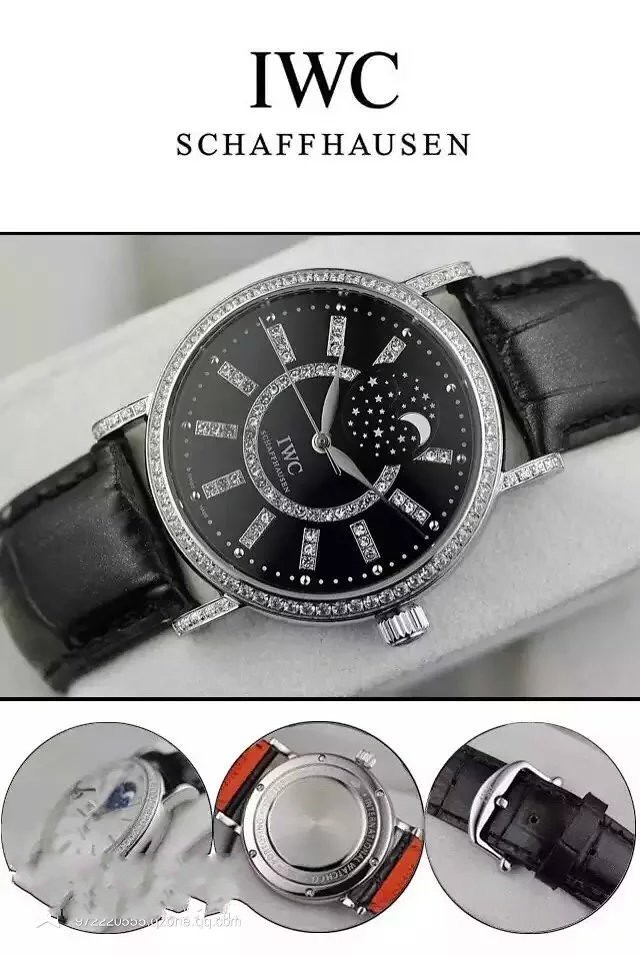**Caption:**

This elegant watch advertisement for IWC Schaffhausen showcases a luxurious timepiece that exudes sophistication and refinement. The main image highlights a watch that appears to be designed for women, featuring a sleek black leather band resting on a light grey watch holder. The watch's edge is silver and adorned with clear, diamond-like crystal jewels. The minimalist dial is emblazoned with the IWC Schaffhausen logo and eschews traditional numbers in favor of a radiant sunburst pattern, with each ray marking the hours. At the 12 o'clock position, a charming subdial displays a moon and stars, adding an element of celestial beauty.

Below the primary image, the ad provides detailed close-ups of the watch's various features. The leftmost image, though slightly obscured by a black smudge, gives a partial view of the watch's side and face. The center image offers a glimpse of the meticulous craftsmanship on the back of the watch, while the rightmost image highlights the polished watch buckle. Together, these detailed visuals emphasize the blend of timeless elegance and modern design that defines IWC Schaffhausen's exceptional craftsmanship.